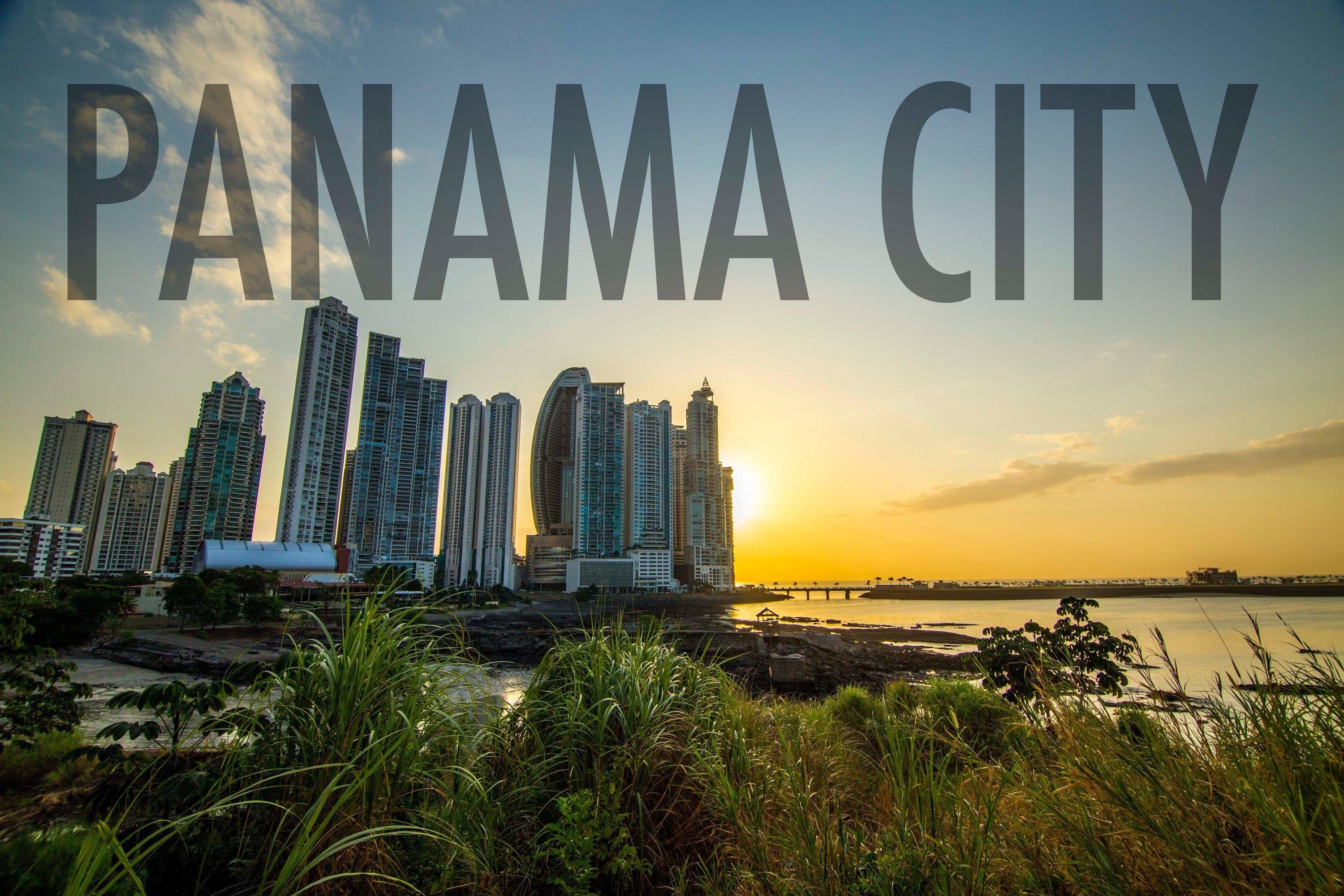An image of Panama City captures a serene yet vibrant scene at sunset. At the top, the words "PANAMA CITY" are inscribed in all capitals with a low opacity gray, giving them a sort of transparent look. The text is uniformly justified with all characters maintaining the same height and width. To the top left, a delicate, wispy white cloud floats against a sky that transitions from pastel light blue to a very light sky blue. 

In the center of the image, the setting sun dominates, casting a bright glow that tapers off into a softer yellow, signaling the end of the day. On the left side of the image sprawls a cityscape, showcasing several tall, rectangular buildings. One building on the right side stands out with two oval-shaped structures, while another nearby boasts a curved design with copper accents.

A calm body of water stretches across the scene, punctuated in the background by a bridge with three supportive pillars. The bridge features an opening on the far left, likely for the passage of ships. Surrounding the city's base and leading into the water are numerous flat rocks.

In the foreground, lush green vegetation mixed with patches of beige—indicating less healthy areas—dominates the scene. The area is interspersed with dark and light green grass. Within this tableau, a couple of vehicles are visible: a semi-truck, possibly carrying a water tank, and another vehicle near a building foundation that appears grated.

This enchanting portrayal of Panama City at dusk underscores the harmonious blend of urban and natural beauty.